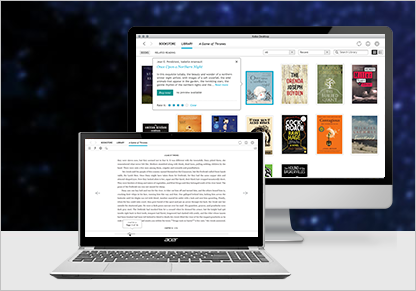A photograph captures a workstation setup, focusing on a computer monitor and a nearby laptop. The monitor, positioned in the background, features a sleek pedestal base that curves elegantly to support it above the desk. The display shows a website with various book images, and a teal-colored pop-up window is visible on the screen. The background of the monitor's screen transitions from a sparkling navy in the upper right corner to a darker shade in the lower left. In the foreground, slightly to the left of the monitor, a Chromebook or laptop rests on the table. The laptop's screen shows a document with several paragraphs, suggesting the user might be engaged in writing or editing a text in a program such as Google Docs. The overall ambiance of the workspace is functional and tech-savvy, highlighted by the digital content displayed on both devices.